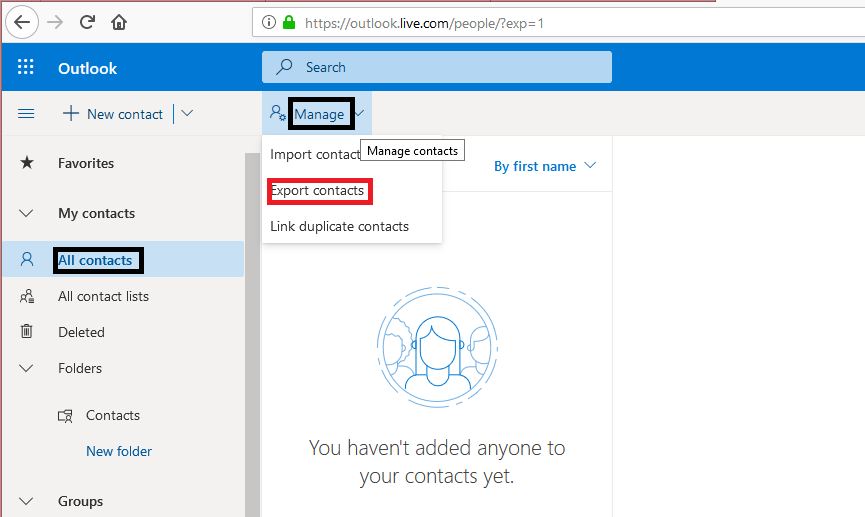The image depicts the "All Contacts" page within an Outlook online portal. On the left side of the screen, there is a vertical menu, with one of the options highlighted in light blue, labeled "All Contacts," indicating that it is currently selected. This option is bordered by a black square. 

The main window on the right side of the screen shows various contact management options. At the top, the "Manage" button is also bordered by a black square. Directly below it, options such as "Import Contact" and "Manage Contacts" are visible. The "Manage Contacts" option is followed by a dropdown menu indicated with a downward arrow, suggesting sorting options by the first name.

Another highlighted option, bordered by a red square, is labeled "Export Contacts." Below the export option, there is a link for "Link Duplicate Contacts," which helps users manage and merge duplicate contact entries. At the bottom, there is a circular icon with a silhouette of a person in the center, possibly representing a button to add a new contact or user profile.

Overall, the interface is designed to manage and organize contacts efficiently within the Outlook online portal.